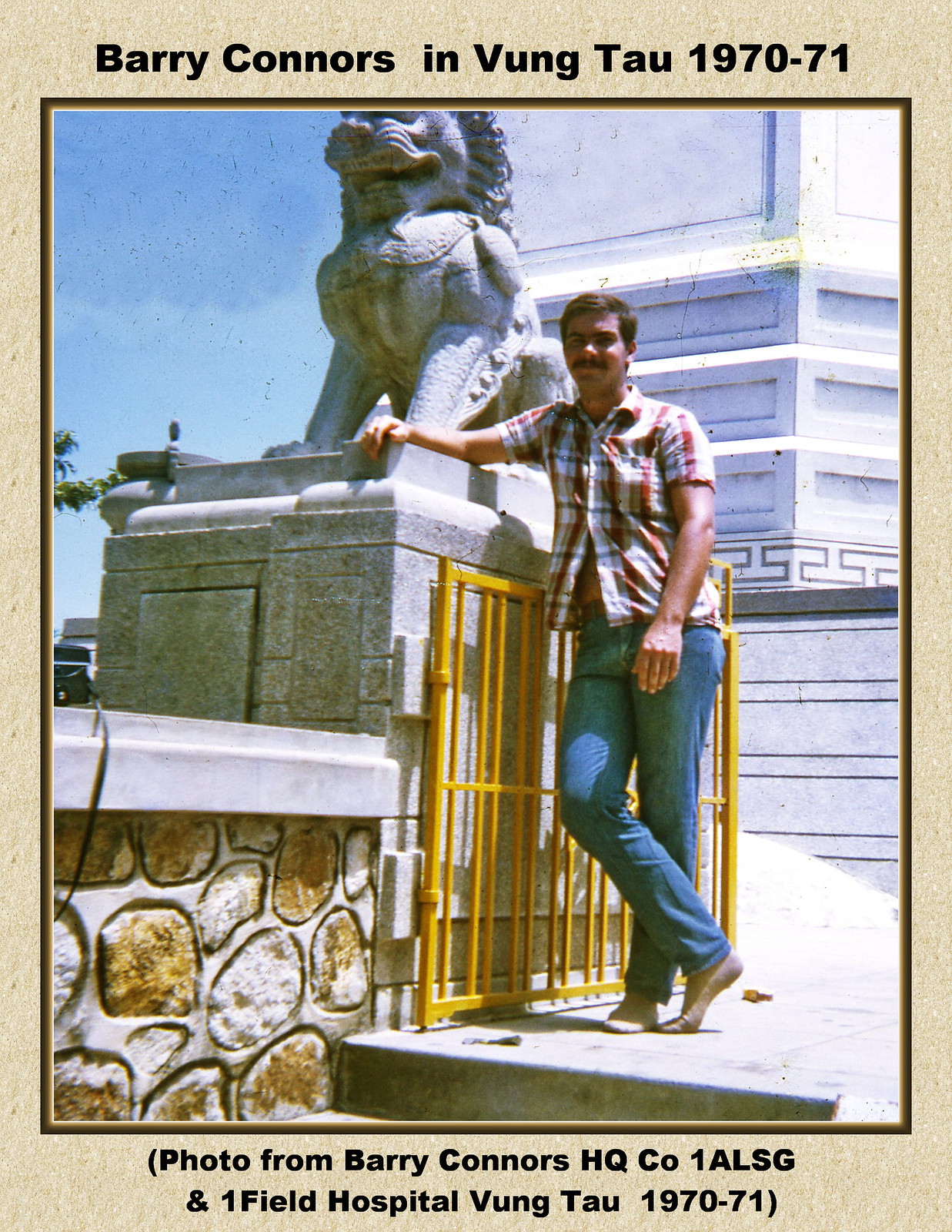The image is a tall, rectangular photograph encased in a digital frame with a beige textured border and an inner frame of a browner, thicker line. At the top, in bold black font, the caption reads "Barry Connors in Vung Tau 1970-71." The bottom caption, also in black font, reads "(photo from Barry Connors HQ Co. 1 ALSG and 1 Field Hospital, Vung Tau 1970-71)." The photograph captures a Caucasian man, identified in the captions as Barry Connors, leaning against a large, ferocious-looking stone lion statue. Barry stands on the bottom step of a cement staircase, wearing a white and red plaid short-sleeved shirt, unbuttoned at the bottom, revealing a bit of his stomach, tight blue jeans, and white socks, with no shoes. His right arm rests on the base of the lion statue, which sits on a substantial cubic gray platform. The lion faces the top left corner of the image, although its head is cut off. Behind Barry, a large white structure is visible, along with a yellow gate to his left. Adjacent to the statue, there is a stone wall with a white top, composed of inlaid brown and white stones.